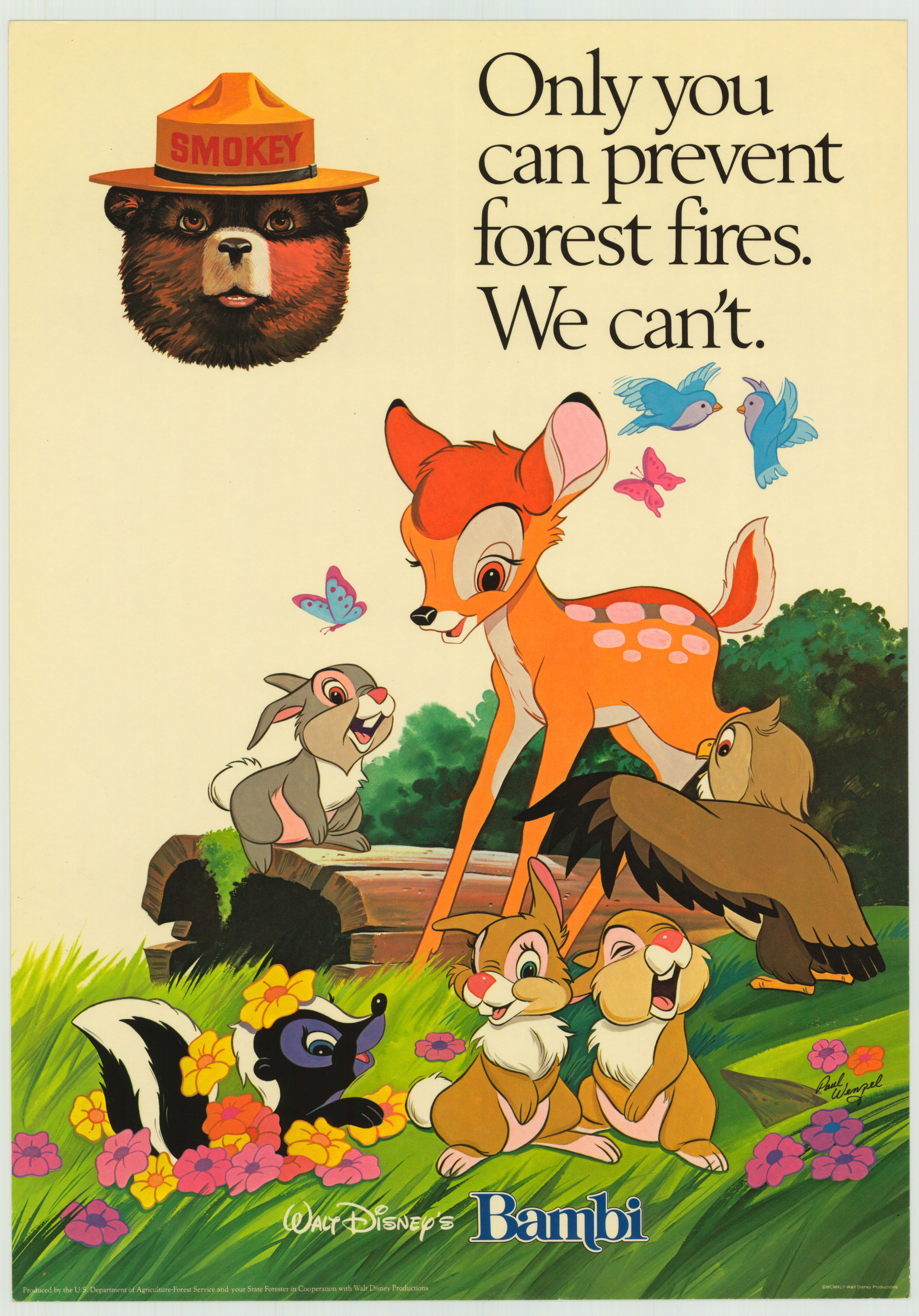This vertical, beige-colored promotional poster from the U.S. Forest Service prominently features the famous Smokey the Bear at the upper left corner, wearing his signature ranger hat with "Smokey" inscribed in red letters. The bold, impactful message atop reads, "Only you can prevent forest fires. We can't," emphasizing the role of individuals in fire prevention. The bottom two-thirds of the poster showcases a vibrant scene from Walt Disney's "Bambi." On the right, Bambi stands gracefully, gazing downward towards Flower the skunk, who is adorably nestled in a bed of multicolored flowers and smiling directly at the viewer. Surrounding them, a lively setting includes blue bluebirds and pink butterflies fluttering about. Thumper the rabbit is perched on a tree trunk behind Bambi, looking up with a cheerful expression. Additionally, there are two brown and white bunny rabbits in the foreground, and an owl is also visible, adding to the forest charm. At the bottom, the text reads "Walt Disney's Bambi," highlighting Disney's collaboration on this engaging and educational advertisement.